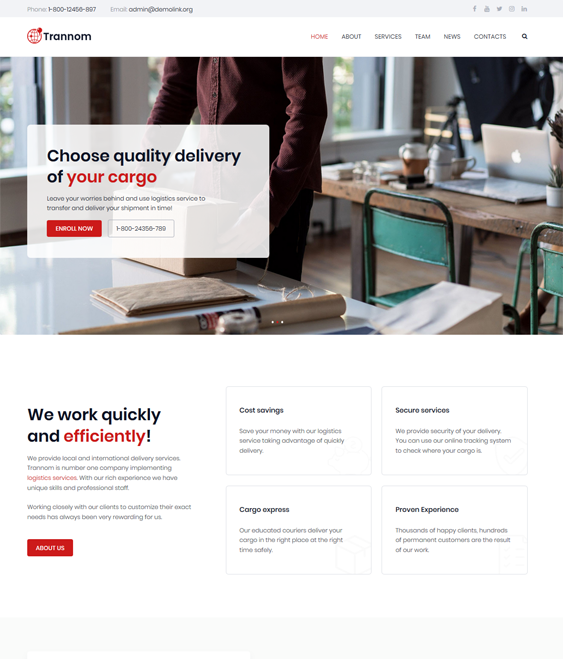This detailed descriptive caption for the webpage image captures all the key elements:

---

The webpage layout is designed for computer viewing. At the top, there is a contact section featuring a phone number and an email address ending in ".org." The exact email is unclear. On the upper right corner, social media icons for Facebook and Twitter are visible. Beneath these icons, a white bar stretches across the page, displaying a red globe symbol with a pinpoint marker and the business name "TRANOM" in black text.

The navigation menu includes categories such as Home, About, Services, Team, News, Contacts, and a search icon. Below the navigation menu, a large, vibrant image occupies about half of the page. The scene is bright and sunny, showing a wooden desk and some retro aqua-blue metal chairs. A person stands next to the desk, wearing a dark burgundy button-down shirt and dark pants. He is wrapping a box with string on a glossy white table, which also has other wrapping materials on it.

Behind him, on the wooden desk, there is a laptop, a couple of coffee mugs, and additional equipment. The background features two large windows and a white wall. Below the image, there is a caption that reads "Choose quality delivery of your cargo" with "your cargo" highlighted in red. Another section says, "Leave your worries behind and use logistics services to transfer and deliver your shipment in time," accompanied by a button labeled "Enroll Now" and a clickable phone number.

Further down, a text reads, "We work quickly and efficiently," followed by an "About Us" section, which can be clicked for more information. To the right, four main points are listed: Cost Savings, Secure Services, Cargo Express, and Proven Experience, though the text is relatively small.

---

This description provides an accurate representation and clear understanding of the webpage layout and its contents.